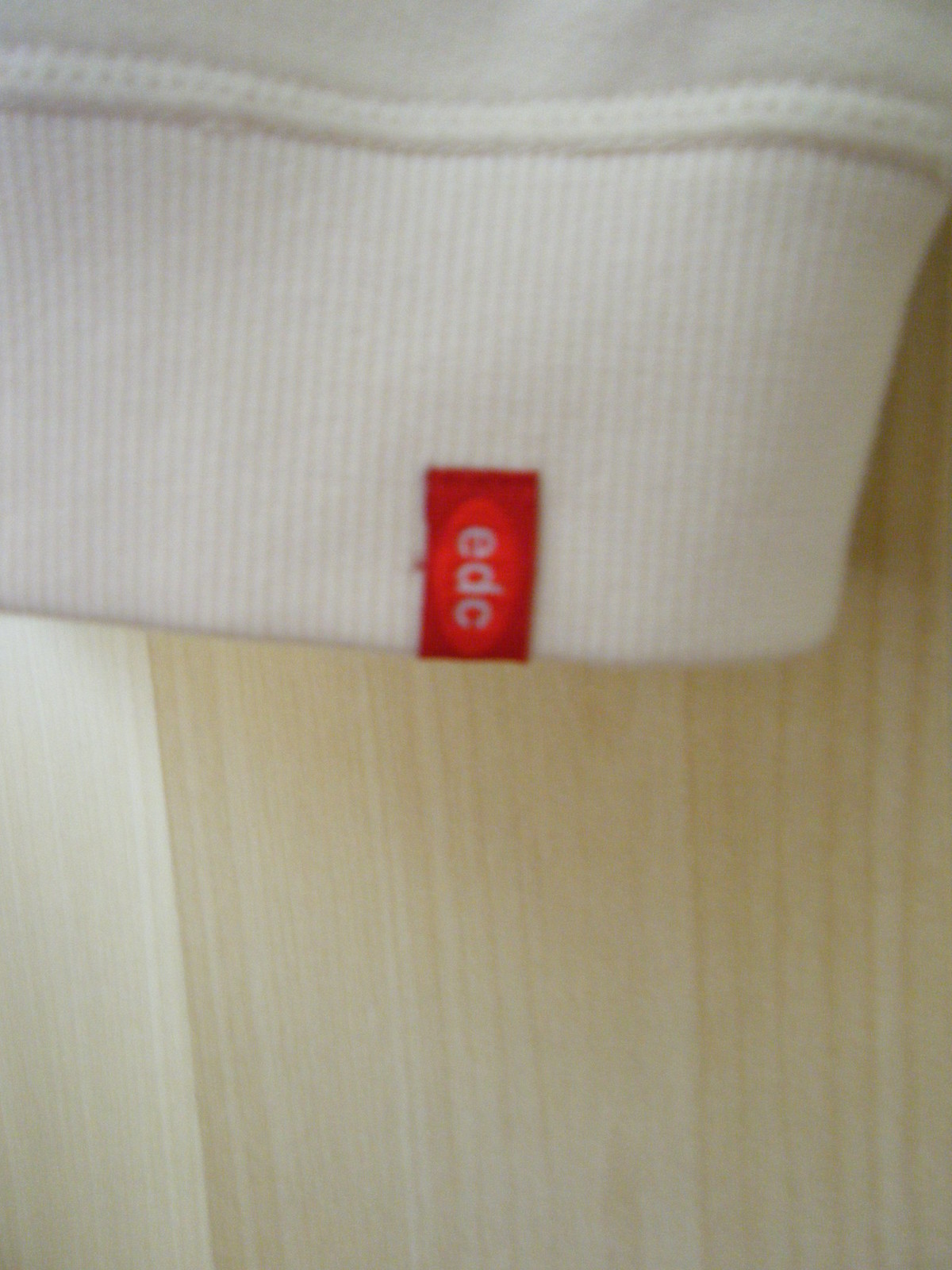This photograph captures a close-up of the bottom hem of a piece of clothing, prominently showcasing its detailed craftsmanship. The hem features a horizontal seam at the top, followed by a section with vertical seams running downwards, highlighting the garment's meticulous stitching. Attached to the hem is a distinctive, rectangular red tag adorned with a lighter red oval and silver lettering that reads "EDC." The background sets off the clothing item beautifully, composed of light tan, almost white wooden panels with vertical grain patterns in varying shades, providing a rustic yet elegant contrast to the vibrant red tag.